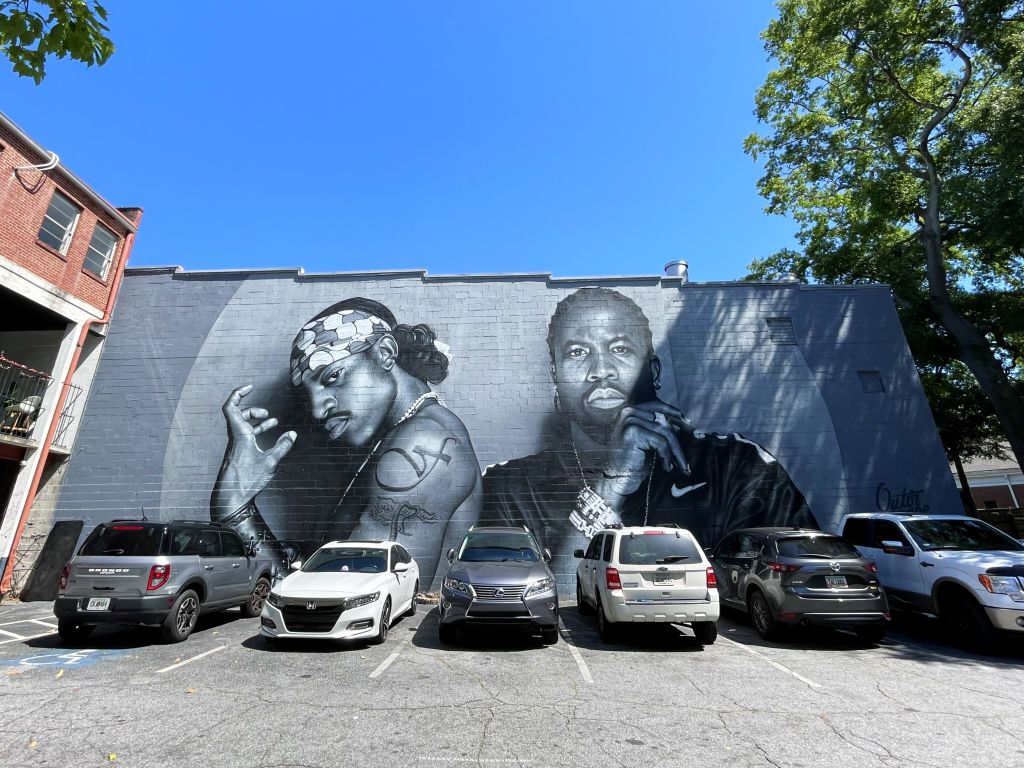This vertical, rectangular image showcases a vibrant mural painted on a gray wall behind a parking lot filled with six cars of varying colors including gray, white, and black. The mural prominently features two African-American men who bear a striking resemblance, possibly indicating they are the same person depicted in different styles or poses. The man on the left, who has a muscular build and a tattooed arm, is seen holding his hand in an unusual gesture and wearing a bandana over his forehead. The man on the right wears a suit coat adorned with a Nike logo, and has hair braids along with a mustache.

In the foreground, the parking lot is lined with parked cars, some facing forward and some backward, adding to the urban atmosphere of the scene. On the left side of the image, there is a slanting, A-frame building with a silver roof and numerous windows. This red building is complemented by a tree with lush foliage, juxtaposed against a bright blue, cloudless sky. The background adds to the image, showing what appears to be an apartment building with peach-colored walls, columns, and chairs placed on a second-story deck.

The mural appears to commemorate iconic figures André 3000 and Big Boi of the musical duo OutKast, with André 3000 depicted shirtless and sporting tattoos while holding a mic, encapsulating elements of their distinctive and influential style.